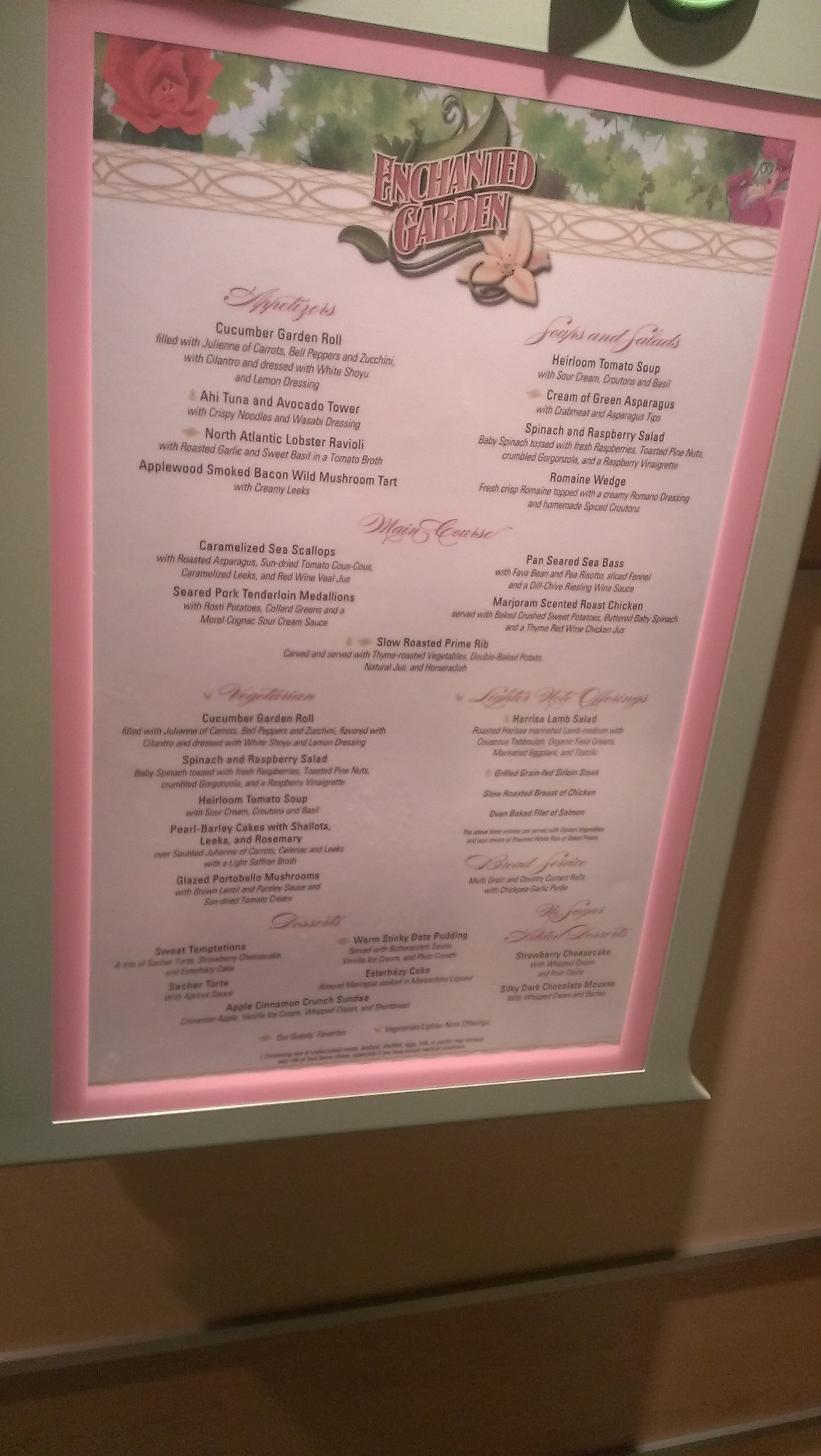This photograph captures a meticulously framed menu situated at the entrance of an elegant dining establishment. The top of the menu features a captivating logo set against a lush floral and green leaf backdrop, reading "Enchanted Garden" in pink letters. Above the menu is a delicate line of greenery complemented by a pink flower image on the left side. The menu sections are clearly marked, showcasing appetizers, soups, salads, and main courses. As the viewer's gaze moves downward, the print becomes increasingly blurry, making some parts difficult to read, though "desserts" is faintly discernible among the entries.

Highlighted dishes include a refreshing "Cucumber Garden Roll," a rich "Heirloom Tomato Soup," and luxurious "Caramelized Sea Scallops." There is also mention of "Pan-Seared Sea," but the type of fish cannot be identified. Additionally, the menu boasts a "Roasted Chicken" and an array of delectable rolls, suggesting a variety of high-end culinary options. The menu exudes sophistication, framed in a light pink color and affixed to the wall. It is elegantly illuminated from above by a spotlight, enhancing its attractive presentation.